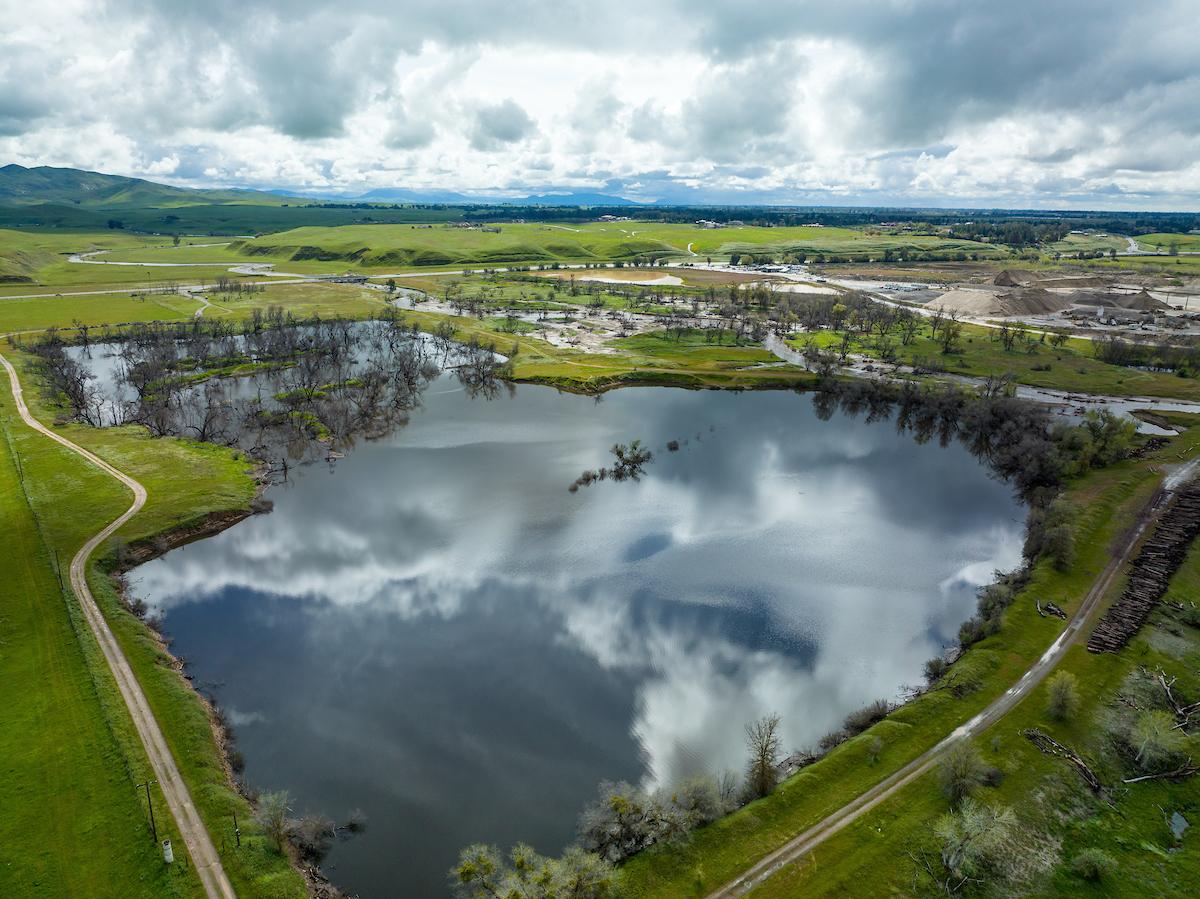This vibrant aerial photograph features a large, almost heart-shaped lake with a distinct circular section at the bottom and a more squared-off region at the top. The lake, with its glass-like surface, perfectly mirrors the stormy sky above, with clouds of white, gray, and patches of cyan blue. Scattered within the lake and along its banks are numerous leafless, brown trees and small island-like patches covered in green grass. There is also a small central island adorned with green foliage.

Encircling the lake is a thin road, beside which lies various natural and man-made elements such as a conspicuous stack of wood, a sand pile, and what looks to be ongoing construction with large mounds of earth and gray-brown pathways. To the right and back of the lake, an evergreen forest stands, creating a lush green backdrop that extends into expansive grasslands.

In the distance, a breathtaking panorama unveils hilly terrains transitioning into towering, green mountains. The scene hints at industrial activity, possibly a quarry or new development, suggesting the lake might be a man-made reservoir. This harmonious blend of nature, human influence, and atmospheric drama paints a vibrant, dynamic landscape.